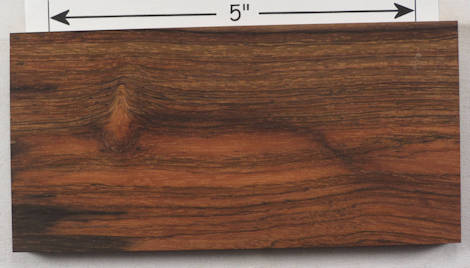This image was taken indoors and features a person measuring a piece of wood. At the top, a white rectangular piece of paper displays black arrows pointing left and right, indicating a length of 5 inches. Below this, the medium brown wood plank, possibly cedar, showcases distinct swirls and black striations. The plank is resting on a gray or white background, likely a table, which emphasizes the reddish-brown hue of the wood as it spans from left to right across the image. The focus of the photograph is the detailed measurement of the wood plank, highlighting its 5-inch length.